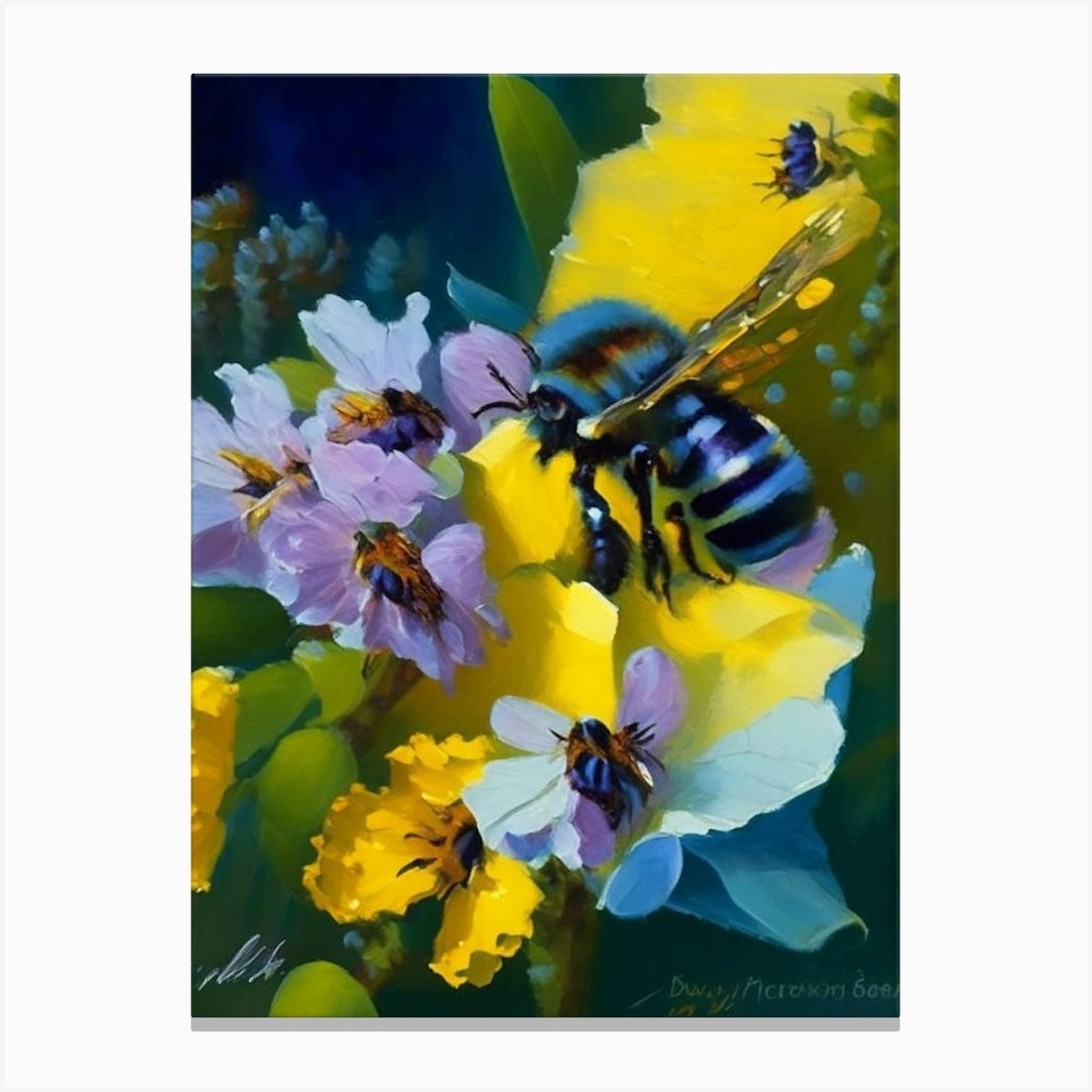This detailed illustration depicts a vibrant scene featuring a cluster of vividly colored flowers, with petals in shades of yellow, lavender, blue, and pastel purple. The background is painted in a deep, dark blue, providing a striking contrast to the bright elements in the foreground. Prominently hovering over and perched on these flowers are a collection of bumblebees, their bodies adorned with alternating stripes of light blue and dark blue, and sporting gold-colored wings. Each bee is rendered in a realistic style, contributing to the overall lifelike appearance of the artwork which incorporates delicate details such as green foliage scattered throughout. There is also some indistinct writing present in the bottom corners of the image.